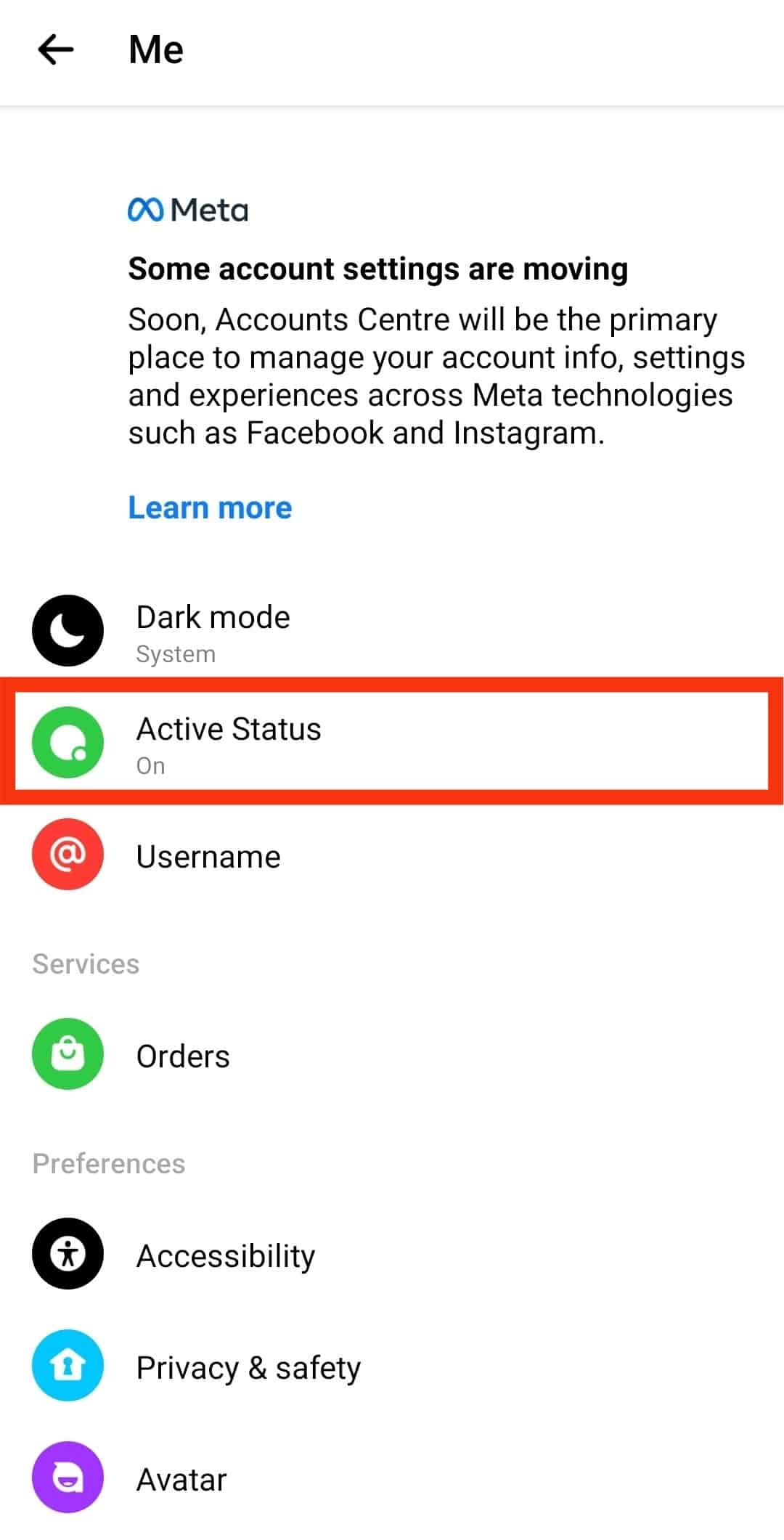In the image, we are presented with a screen from an app, specifically a settings or account management page. 

At the top of the screen, there is a back arrow symbol, accompanied by the text "Me." Directly below this, on a clean white background, the familiar Meta logo is displayed next to the word "Meta."

A prominent message below the logo indicates that "Some account settings are moving." It further explains that the "Meta Account Center" will become the primary location for managing various account details, settings, and experiences across Meta technologies, including Facebook and Instagram. Beneath this explanatory note, there is a "Learn More" button for additional information.

Following this, the page features a series of clickable options, each with a corresponding icon:
1. **Dark Mode** - Represented by a moon icon.
2. **Active Status** - Indicated by a green circle icon.
3. **Username** - Denoted by a red at symbol (@).

The section labeled "Services" follows, presenting additional options:
- **Orders** - Versatile by a purse icon.

At the bottom of the screen, under the heading "Preferences," there are three distinct options:
1. **Accessibility** - Illustrated by a human figure inside a black circle.
2. **Privacy and Safety** - Symbolized by a blue circle with a house icon featuring a keyhole.
3. **Avatar** - Depicted by a purple circle containing an emoji icon.

This detailed structure provides users with a comprehensive range of settings, ensuring easy navigation and management of their account preferences and services across Meta platforms.